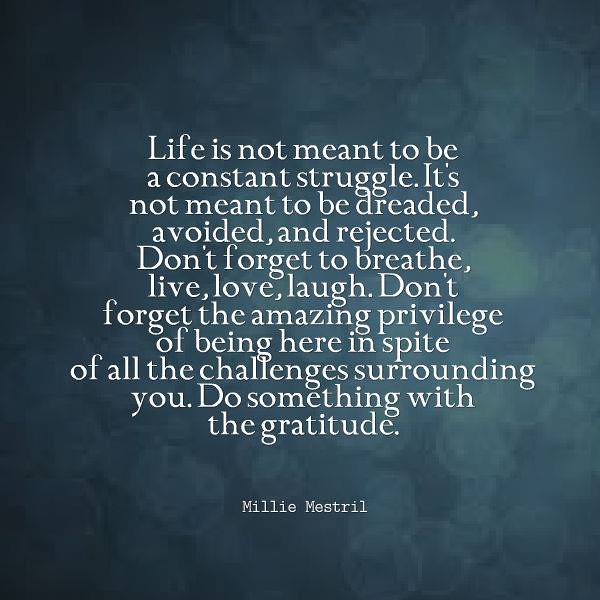The square image features a variegated blue background with a subtle gradient that transitions from a darker blue in the top left corner to a lighter blue as it moves towards the center and lower right. The background also includes delicate circular patterns that resemble blurred raindrop spatters on a window, adding an abstract, out-of-focus effect. Superimposed in the center of this background is an inspirational quote, written in a white, typewriter-like font:

"Life is not meant to be a constant struggle. It's not meant to be dreaded, avoided, and rejected. Don't forget to breathe, live, love, laugh. Don't forget the amazing privilege of being here in spite of all the challenges surrounding you. Do something with the gratitude."

A few spaces below the quote, in a smaller font and also centered, is the attribution: "Millie Mestral." The entire design harmoniously blends the elements of graphic design and typography to create an inspiring visual message.